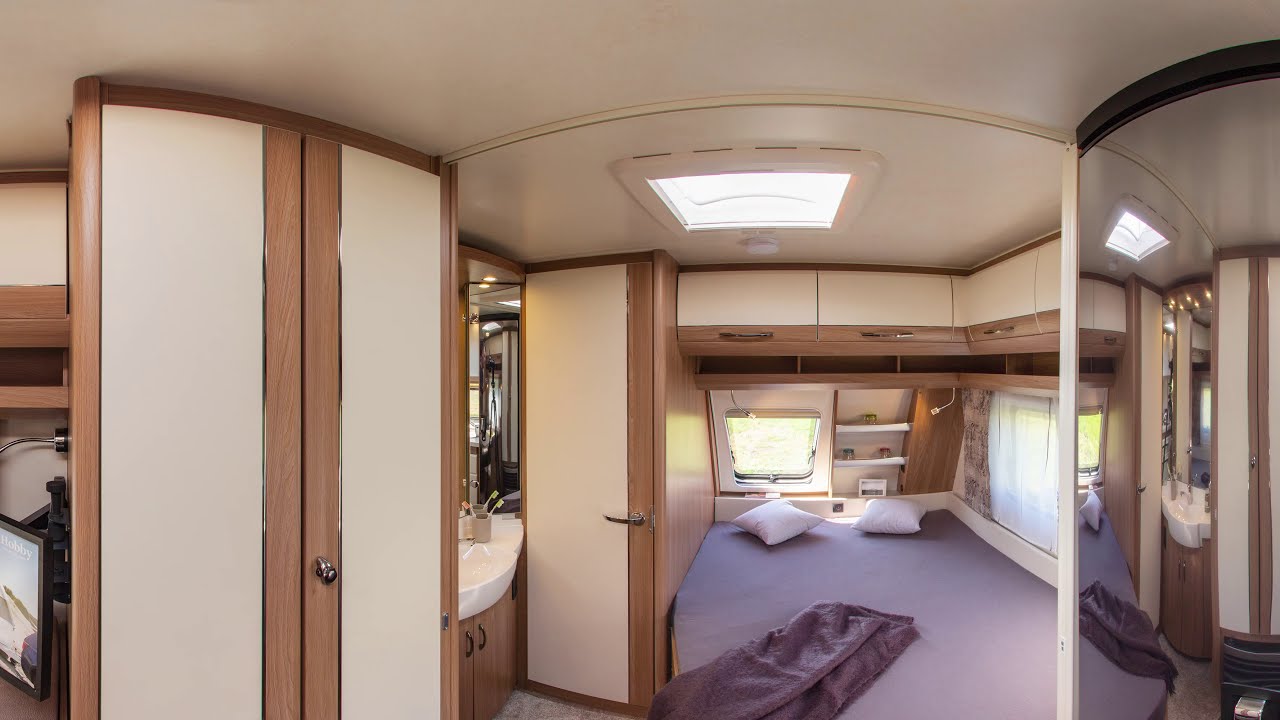The image appears to be taken inside a small, possibly mobile living space such as an RV, camper, or train cabin, during the daytime. On the left side of the image, there is a large, two-door closet with white doors framed with wooden outlines and stainless steel handles. Next to it, slightly to the right and closer to the viewer, there is a smaller closed closet and a sink area with a wooden cabinet and a white vanity top. 

On the right-hand side, a floor-to-ceiling mirror reflects parts of the space, including the sink and contributing to the panoramic view. The bed is positioned along the right wall, flush against it, featuring purple sheets, pillows, and a blanket. Above the bed are storage compartments and a couple of shelves. The wall adjacent to the bed has a large window, providing natural light to the interior, which suggests it’s daytime. Additionally, there is a smaller window next to the bed and a skylight on the ceiling, further illuminating the space. The colors in the image include shades of white, tan, brown, black, and different shades of purple and green, creating a cozy yet compact living environment.